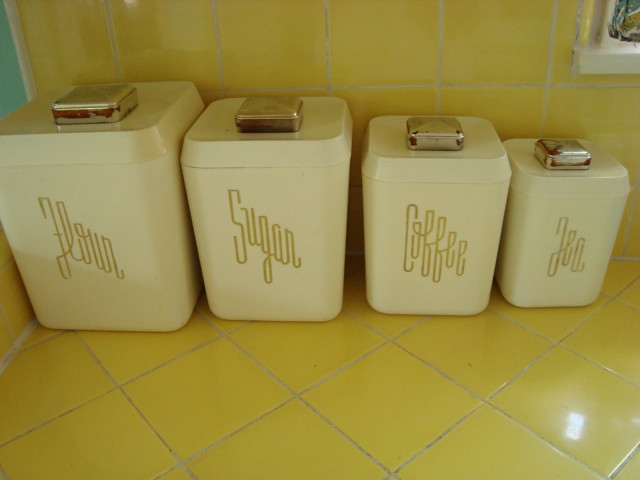This is a detailed color close-up photograph of a yellow-tiled kitchen. The countertop, adorned with yellow diamond-shaped tiles and white grout, perfectly mirrors the wall behind it, which features yellow square tiles. In the right-hand corner of the frame, a small white-painted window adds a touch of brightness to the well-lit room. Against the wall are four vintage-style square canisters of ascending size, from left to right. These canisters, repurposed soap dispensers painted a yellowish cream color, all have silver tops and cursive gold writing on their fronts. The labels read "flour," "sugar," "coffee," and "tea," with the word "flour" placed diagonally beginning at the top left and ending at the bottom right.